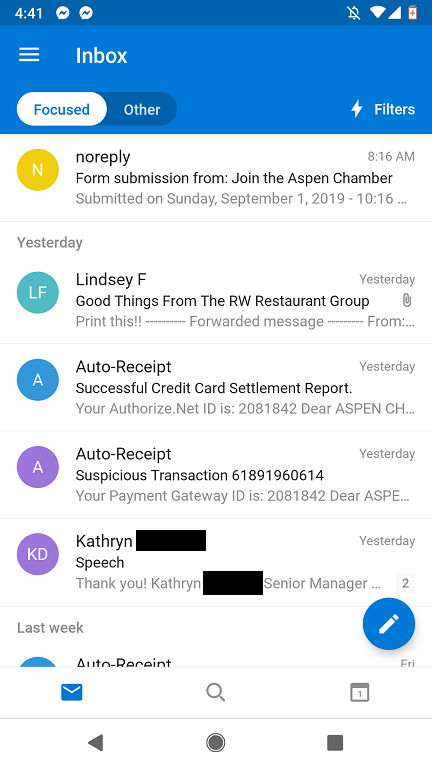This image captures a screenshot of a Gmail inbox interface. At the very top, there is a prominent blue header. The task notification section shows the current time and indicates two unread Facebook Messenger notifications. In the upper right corner, icons display the battery level, cell signal strength, Wi-Fi connectivity, and a muted ringer.

Immediately below the header, there is a navigational bar featuring a list icon, the "Inbox" label, and tabs for "Focused" and "Other" emails. To the right of these tabs is a filters button. The central portion of the image showcases the email list against a white background, with each email marked by a round avatar icon indicating the sender. These avatars display a variety of colors: yellow, teal, blue, two purple, and another blue partially visible at the bottom edge of the screen.

One of the emails at the bottom of the screenshot is from a sender named Catherine, with her last name obscured by a black bar. The email preview reads "Thank you Catherine," with the last name again redacted by a black bar.

At the bottom right corner of the screen, the blue "Compose" button is visible, displaying a white pencil icon. Lastly, the bottom section houses typical Gmail function icons for mail, search, and calendar.